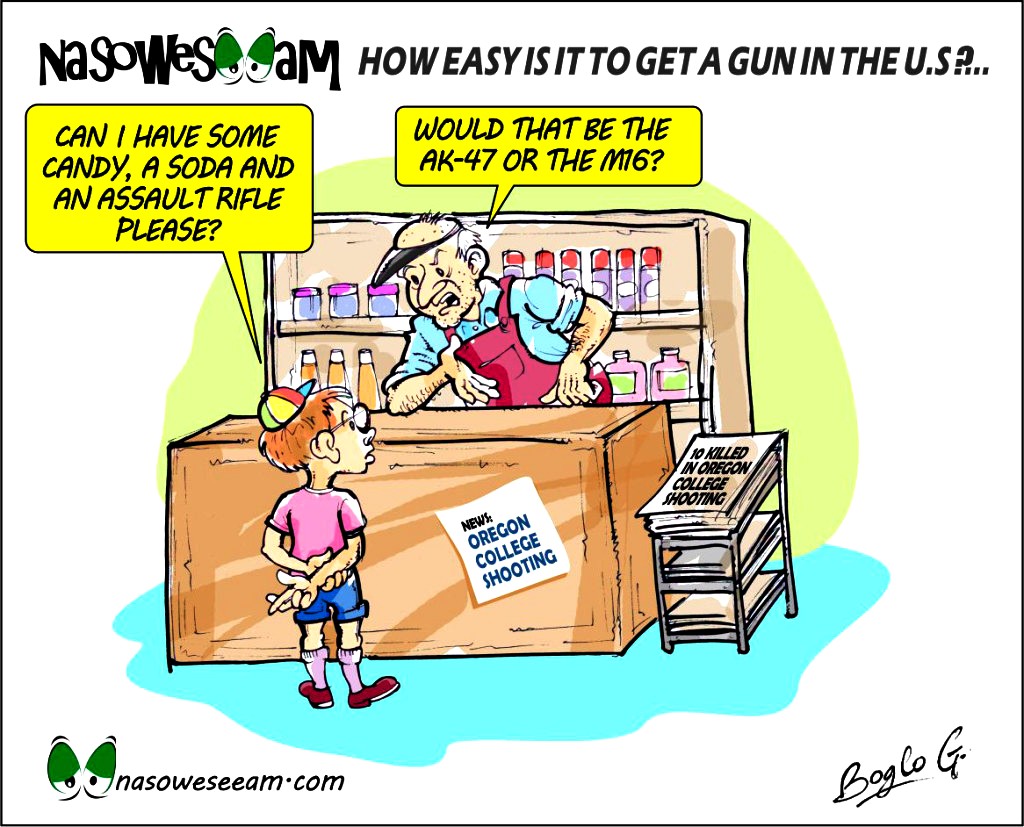This cartoon image titled "NASOWCM" (from nasowcm.com) humorously highlights gun accessibility in the U.S. with a poignant satire. At the top, a caption in a yellow cloud asks, "How easy is it to get a gun in the U.S.?" The scene takes place in a store with a white background, where an old man in a cap and red apron stands behind a counter. The counter is lined with various cans, papers, and a rack of goods. A geeky-looking young boy, wearing glasses, a baseball cap, purple socks and shoes, jean shorts, and a purple t-shirt, approaches the counter. With fingers crossed behind his back, the boy requests, "Can I have some candy, a soda, and an assault rifle, please?" The old man nonchalantly responds, "Would that be the AK-47 or the M16?" On the counter, a newspaper headline reads, "10 Killed in Oregon College Shooting," referencing a tragic event. The lower corner of the image bears the artist's signature, "B.O.G." Two cartoonish eyeballs are also visible in the lower left corner, adding to the image's comedic yet critical tone.